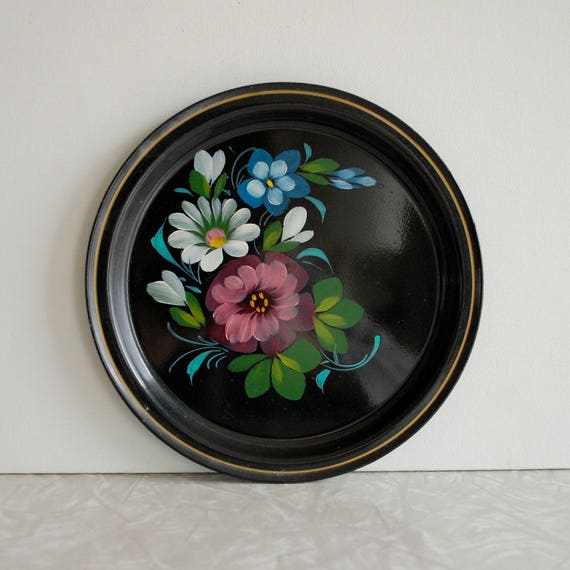The image showcases a detailed scene featuring a decorative plate, prominently displayed against an off-white wall with a tan floor. The plate is circular and black, featuring a goldish-copper rim. Intricately painted in the plate's center is a floral arrangement consisting of three primary flowers: a red flower with petals transitioning from pink to yellow at the center, a white flower with a green transition to a yellow center, and a medium-to-light blue flower also culminating in a yellow center. Accompanying the flowers is an abundance of greenery and additional sprigs incorporating blue elements, creating a lush and vibrant composition. The plate, positioned to capture light reflections, adds a dynamic dimension to its appearance. The entire scene is well-balanced, with shadowing hinting at depth and the absence of size references emphasizing the plate's artistic detail.